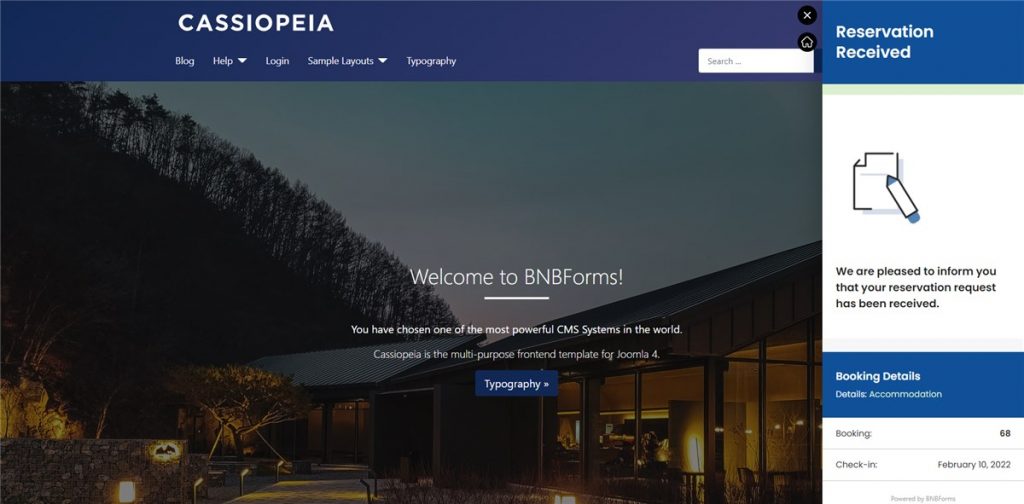Screenshot Description:

The screenshot is taken from a website named "Cassiopeia," as indicated in the top-left corner. Just below the site name, there's a menu bar with options for Blog, Help, Login, Sample Layouts, and Typography, all set against a dark purple background. On the top right, there are an X (close) button, a home button, and a search bar.

The main header below this menu features a generic cabin-like image, overlaid with text that reads, "Welcome to BNB Forms." Under that, smaller text states, "You have chosen one of the most powerful CMS systems in the world. Cassiopeia is the multipurpose front-end template for Jumia 4." There is also a prominent button labeled "Typography."

To the right of this main section, there's a sidebar with a blue background header that says "Reservation Received." Below that, on a white background, the text states, "We are pleased to inform you that your reservation request has been received." The background switches back to blue with the heading "Booking Details," and then returns to white background detailing "Details Accommodation." Further down, it notes "Booking 68, check in February 10, 2022."